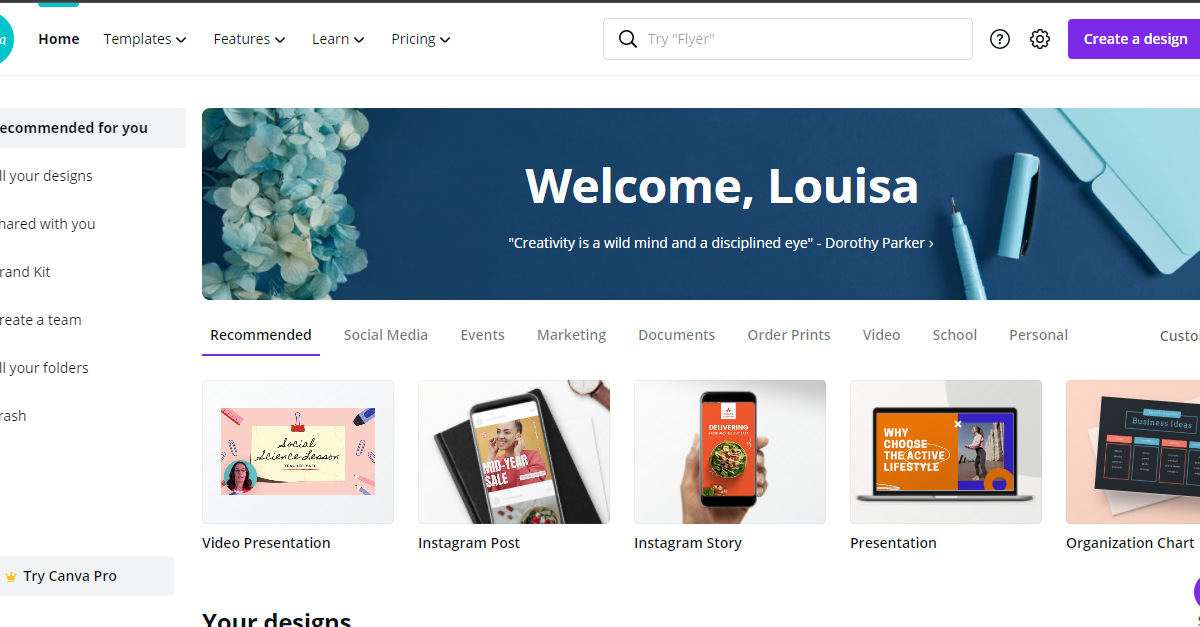The image displays a website interface featuring a predominantly white background. At the top of the page, there is a navigational menu with black text, providing selectable categories such as Home, Templates, Features, Learn, and Pricing. Adjacent to the menu is a search bar with the placeholder text "try flyer." To the right of the search bar are icons for help (a question mark) and settings (a cogwheel), along with a prominent purple button labeled "Create a Design" in white text.

On the left side of the screen, a slightly cut-off sidebar lists various categories: Recommended for You, Your Designs, Shared with You, Your Folders, and Trash. Additionally, there's a suggestion to "Try Canva Pro."

A blue banner spans the width of the page, welcoming a user named Louisa with the inspirational quote, "Creativity is a wild mind with a disciplined eye" by Dorothy Parker. This banner is adorned with a blue pen and file folder graphic to the right, and a blue and yellow floral design to the left.

Below the banner are several categories and sections labeled with text and icons, including Video Presentation, Instagram Post, Instagram Story, Presentation, and Organization Chart. Further down, there is another section categorizing content into groups such as Recommended, Social Media, Events, Marketing, Documents, Order Prints, Video, School, and Personal.